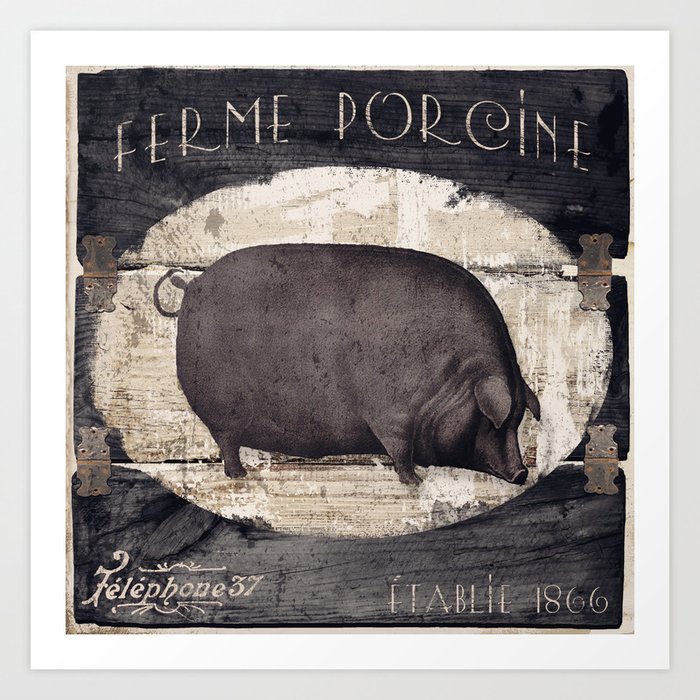In this detailed, monochromatic artwork designed to appear antique, we see a large, rotund pig with a massive body and tiny legs, standing with its head lowered as if sniffing something. The snout is relatively small, and two ears are visible. The entire image is enclosed within an oval shape formed by three pieces of wooden slats, held together by latches and hinges that suggest the setting might be a wooden door. The background wood further complements the old-fashioned aesthetic of the piece. Text written in uppercase letters at the top reads "FERME PORCINE," likely indicating a French term related to pig farming. Beneath the pig, on the lower left, it says "Telephone 37" in cursive, and on the bottom right, "Établi 1866" in all caps, signifying "Established 1866". The pig itself is depicted in dark tones, contrasting with the lighter, perhaps dirt-smeared background around it, enhancing the rustic and vintage feel of the artwork.